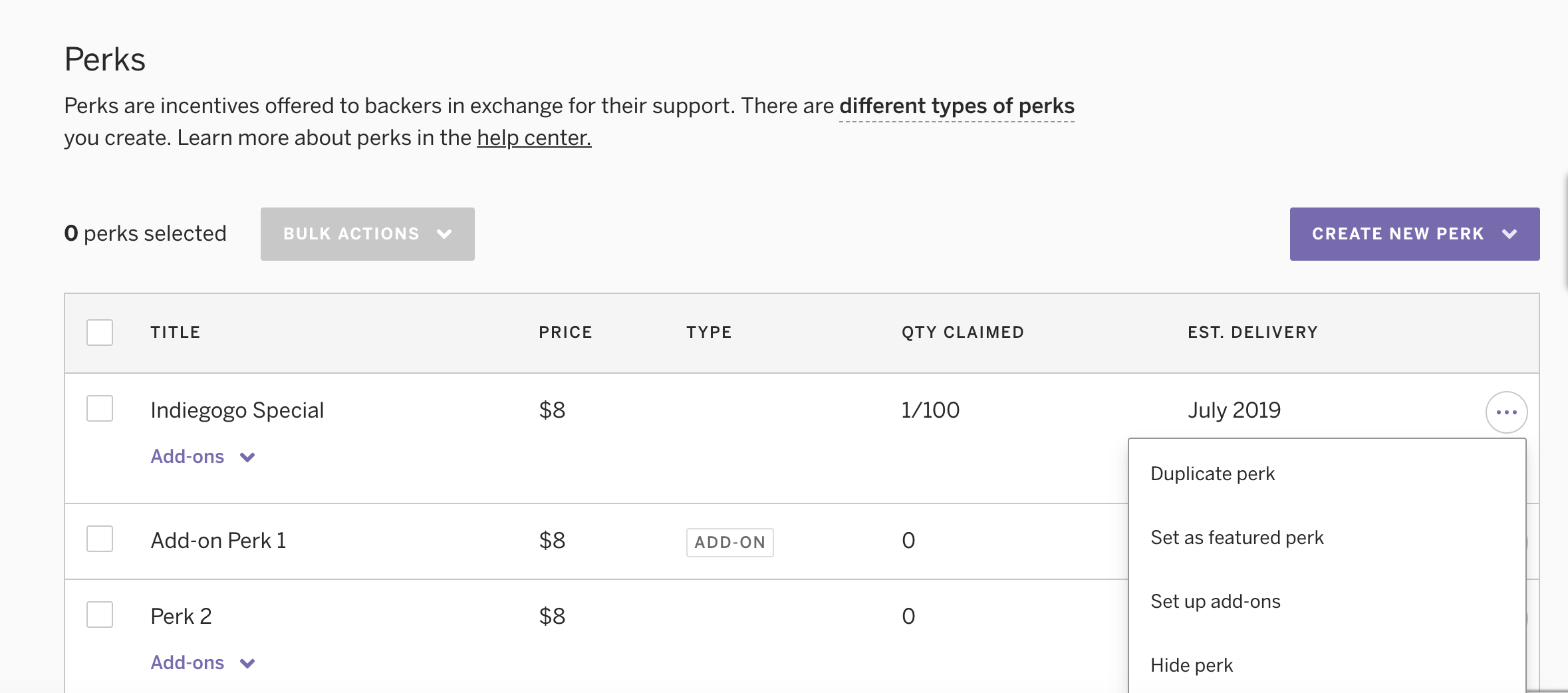The image showcases a web page that features a section dedicated to managing backer perks. In the top left corner of the page, the word "Perks" is prominently displayed against a grayish off-white background, with black lettering. Beneath this heading, there's an explanation: "Perks are incentives offered to backers in exchange for their support. There are different types of perks you can create. Learn more about perks in the Help Center."

Below this introductory text, it reads, "Zero Perk Selected." Adjacent to this, there is a "Bulk Actions" button, and on the far right, a button labeled "Create New Perk."

A table is presented below these elements. The table headers are as follows: "Title," "Price," "Type," "Quantity Claimed," and "Estimated Delivery."

The first row of the table details:
- Title: Indiegogo Special
- Price: $8
- Type: (blank)
- Quantity Claimed: 1 of 100
- Estimated Delivery: July 2019

The second row describes:
- Title: Add-On Perk 1
- Price: $8
- Type: Add-On
- Quantity Claimed: 0

The third row lists:
- Title: Perk 2
- Price: $8
- Type: (blank)
- Quantity Claimed: 0

For both the second and third perks, the "Estimated Delivery" column is obscured by a white box. This box contains options including "Duplicate Perk," "Set as Feature Perk," "Set Up Add-Ons," and "Hide Perk."